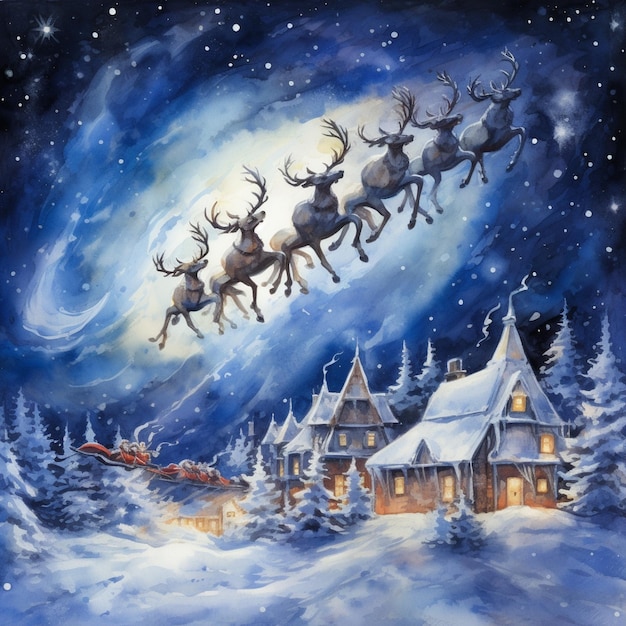This image, likely an AI-generated painting due to some anatomical inconsistencies in the reindeer, depicts a nostalgic Christmas scene. The composition is rectangular, slightly taller than wide, with six brown reindeer flying in a diagonal row toward the upper right-hand corner. These reindeer are inconsistently rendered with between two and eight legs each, suggesting the artwork's digital origins.

Behind the reindeer, the sky transitions from a light blue near the horizon to a deep, star-filled night sky, with a swirling white nebula adding an ethereal touch. High in the sky, scattered round white dots imitate falling snowflakes, enhancing the festive atmosphere. The lower portion of the painting features a snow-covered village with tall, peaked roofs and warm, orange light glowing from the windows. Nestled among the snow-laden pine trees, the buildings, which are constructed from brown brick or wood, exude a cozy and cheerful vibe. Additionally, a disconnected red object resembling Santa's sleigh hovers in the left lower portion of the image, further emphasizing the digital or imaginative style of the painting.